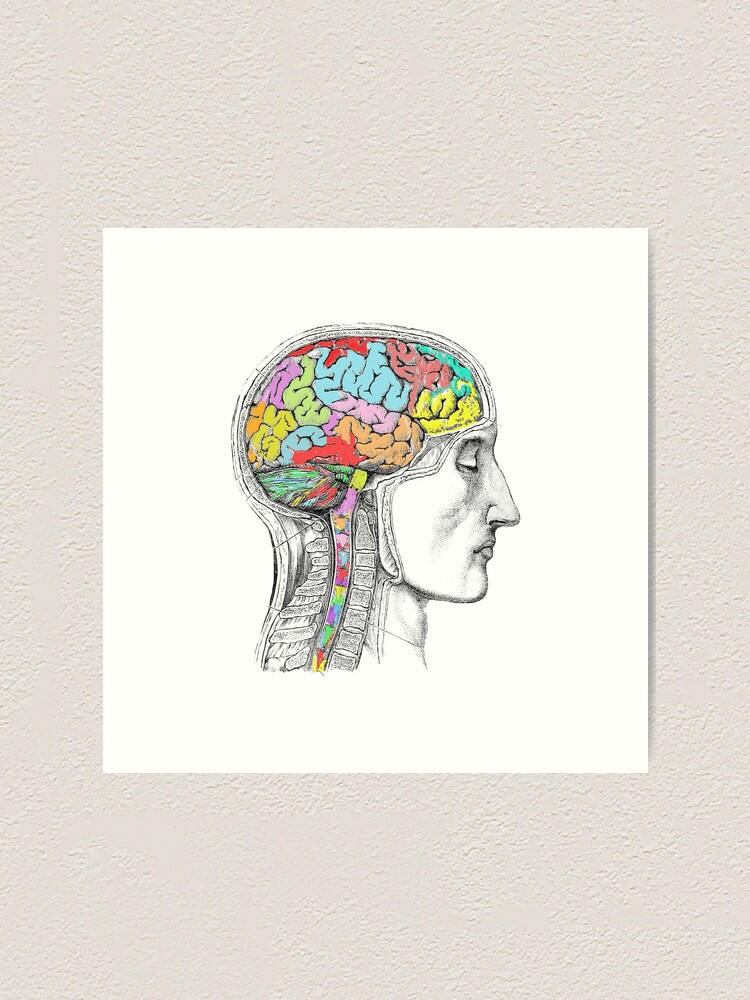The artwork is a detailed, vertically aligned rectangular illustration mounted on an off-white, textured wall. The focus of the piece is a male figure's profile, specifically the right side of his face and neck, depicted in black and white. The figure's eyes are closed, with visible outlines of his nose and lips. The artwork presents an anatomical cut-away, revealing the brain with multi-colored sections in shades of blue, light purple, red, brown, yellow, green, pink, and orange. These colors highlight different brain areas, which extend down into the spinal cord, illustrating signals traveling along the vertebrae. The drawing is on a square white canvas, reminiscent of a medical pencil sketch, complete with lines that suggest labels for various anatomical parts. The surrounding wall has a textured, drywall appearance, adding a subtle contrast to the intricate central piece.